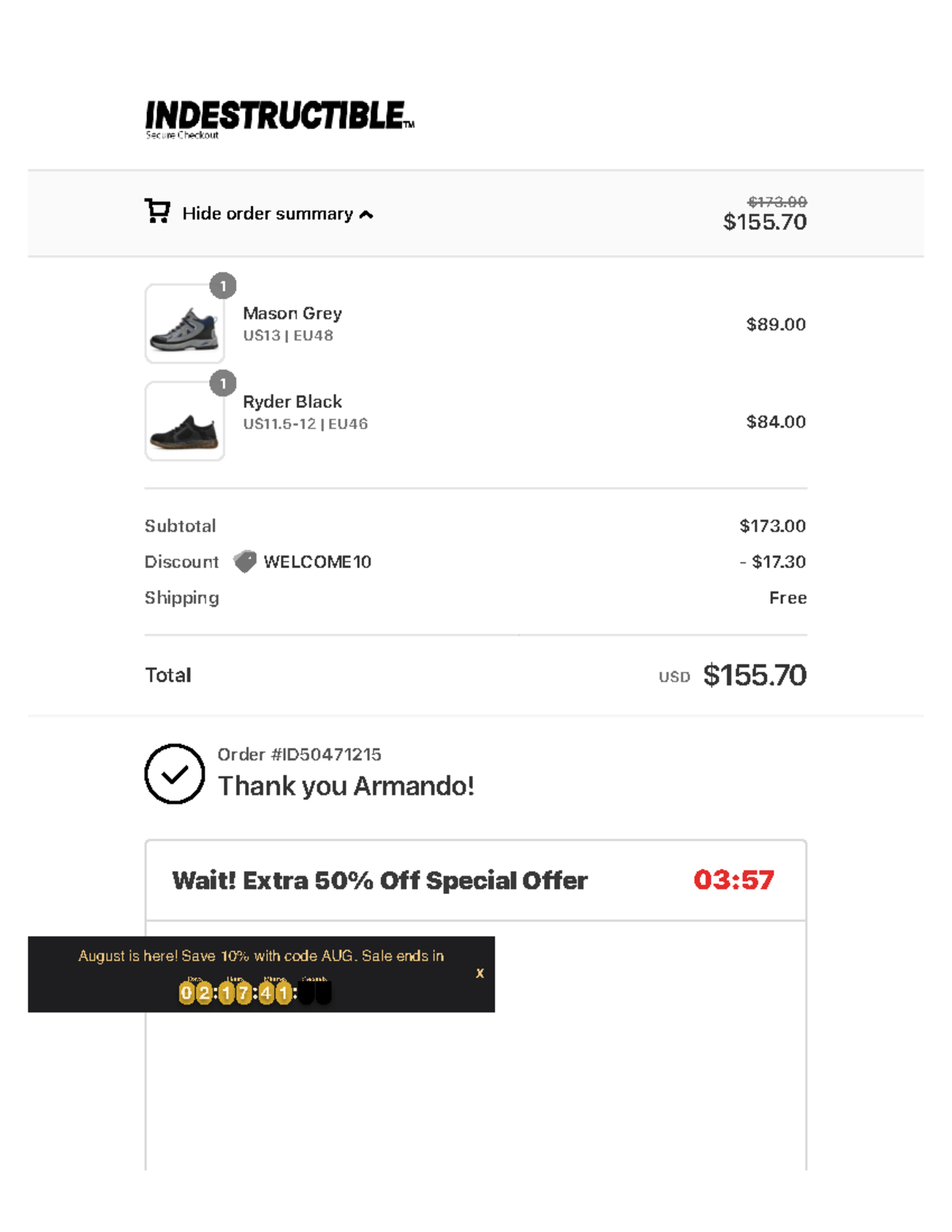The image showcases the checkout page of a website named "Indestructible," featuring a secure and user-friendly interface. On the order summary, a customer named Armando has placed an order for two items. The first item is a pair of Mason Grey training shoes, listed as catalog number US 13 (EU 48) and priced at $89. The second item is a pair of Rider Black training shoes, with a catalog number of US 11.5 to 12 (EU 46), priced at $84. A welcome discount of $17.30 has been applied to the order, and free shipping is included, bringing the total amount to $155.70. The order is identified by the number ID 50471215. Additionally, a special offer is presented, granting an extra 50% off if Armando responds within the next 3.57 minutes.